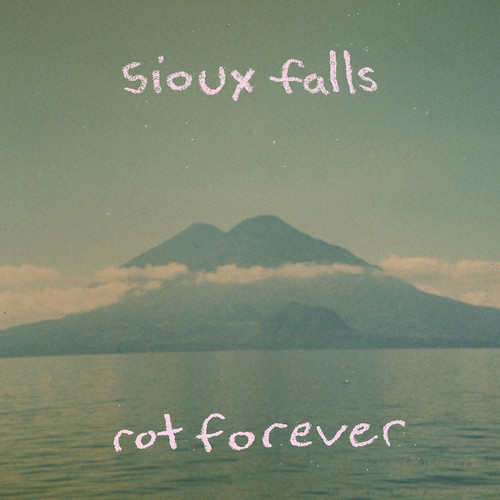This photograph depicts a dim, somewhat unclear scene primarily featuring a large mountain that resembles a volcanic island, encircled by a dark greenish ocean. The mountain or island rises sharply from the water in a triangular shape, with its peak piercing through a low level of white cumulus clouds. The entire image, including the sky and water, is suffused with a greenish hue, making it difficult to discern the true colors of the landscape. The night sky is dotted with numerous stars, adding a mystical aura to the scene. At the top of the image, in white handwritten chalk-like font, reads "Sayuk's Falls," while the bottom bears the similarly styled text, "Rot Forever." The overall graininess and overcast or smoky appearance lend a mysterious, almost eerie quality to the photograph.